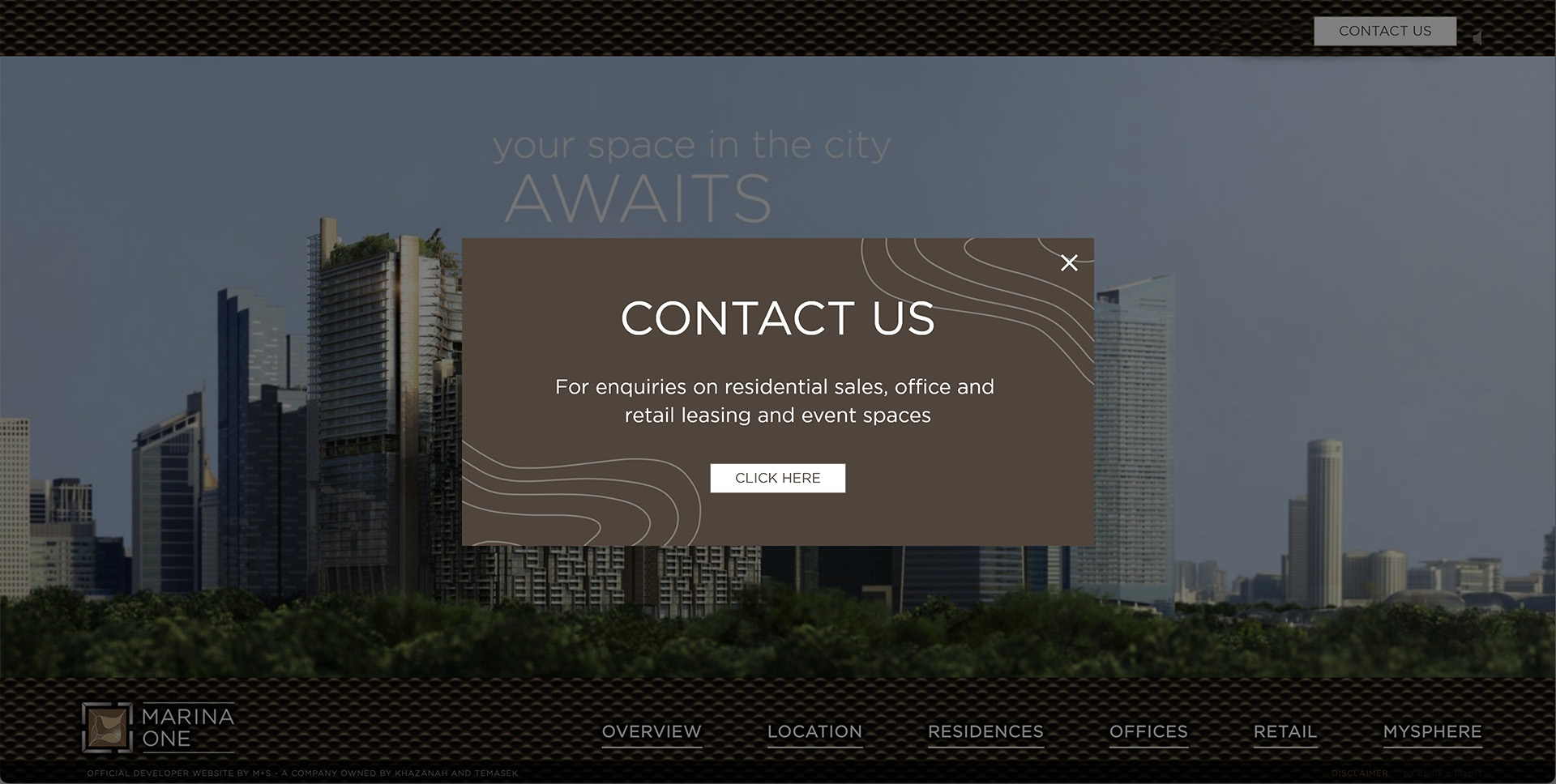This is an image of Marina One's "Contact Us" webpage. The page features black bars with a tire tread pattern paired with gray highlights at both the top and bottom sections. A gray button with "CONTACT US" in bold uppercase black text is situated in the upper right-hand corner. Dominating the main background is an impressive downtown cityscape, showcasing numerous high-rise buildings and potential condominium structures. The foreground is lush with dense, albeit not very tall, trees.

Centrally located on the webpage is a pop-up window in gray, prominently displaying "CONTACT US" in uppercase white font. The pop-up provides detailed information for inquiries concerning residential sales, office and retail leasing, as well as event spacing. Just below this text, a white button with "CLICK HERE" in uppercase black font invites user interaction.

Additionally, from the midpoint spanning to the right-bottom section of the page, there are multiple navigation tabs labeled "Overview," "Location," "Residences," "Offices," "Retail," and "MySphere," providing easy access to various sections of the site.